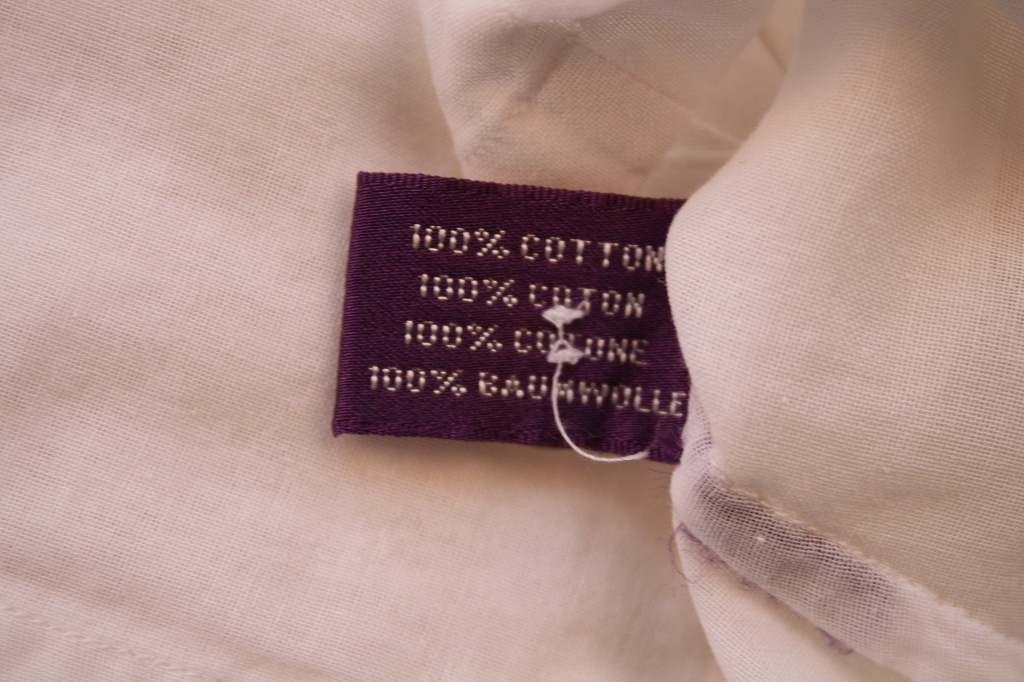The image depicts a close-up of a clothing tag attached to a white or off-white garment, possibly made of linen. The tag itself is black, with white text clearly stating "100% Cotton" in both English and French ("100% Coton"). The tag is fastened in the center of the garment, drawing attention to the material composition. The overall color scheme of the image is minimalistic, dominated by shades of white and black, highlighting the simplicity and elegance of the garment's fabric and the informative tag.